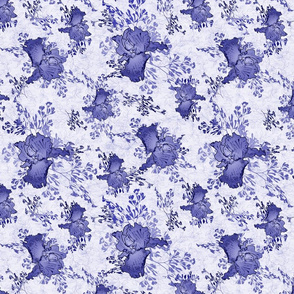The image depicts an intricate, vintage-style wallpaper design that features a repeating floral pattern. The background transitions subtly from a light purple to white, creating a soft, airy ambiance reminiscent of a classic motif you might find in an older home, perhaps your grandmother's. The wallpaper showcases dark navy blue roses, alternatively described as deep purple flowers, accented with leafy designs that give a lush, textured appearance. Each flower is unique in its stage of bloom, with some fully bloomed and others just budding. The pattern is uniformly distributed across the entire square image, with rows of flowers spaced evenly. The larger and smaller flowers are balanced perfectly, each surrounded by delicate purple sprouts or leaves, adding to the detailed, elegant aesthetic of the design.